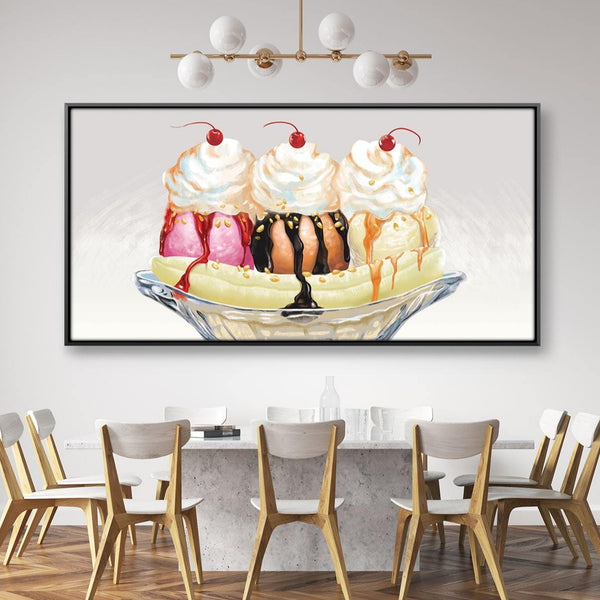The image depicts a modern, stylish interior that appears to be either an ice cream shop or an office space. Dominating the white wall in the background is a large, black-framed painting of a classic banana split sundae, featuring three scoops of ice cream—pink strawberry on the left, caramel-colored chocolate in the middle, and cream-colored vanilla on the right. Each scoop is adorned with its respective syrup—strawberry syrup on the strawberry scoop, chocolate syrup on the chocolate scoop, and caramel syrup on the vanilla scoop—and crowned with a dollop of whipped cream and a cherry. The banana lies horizontally beneath the ice cream scoops in a translucent glass bowl, with a sprinkling of nuts enhancing the sundae's appeal. 

Below this striking artwork is a substantial marble countertop table that can seat about ten people with its sleek, stone surface. The table is surrounded by modern wooden chairs with a minimalist white seat and backrest design. A few glasses, a glass bottle of water, and some books are neatly arranged on the table. The room features hardwood flooring, and hanging from the ceiling above the artwork is a contemporary light fixture comprising six white globe lights attached to a sleek gold rod, casting a warm glow that complements the sophisticated setting.